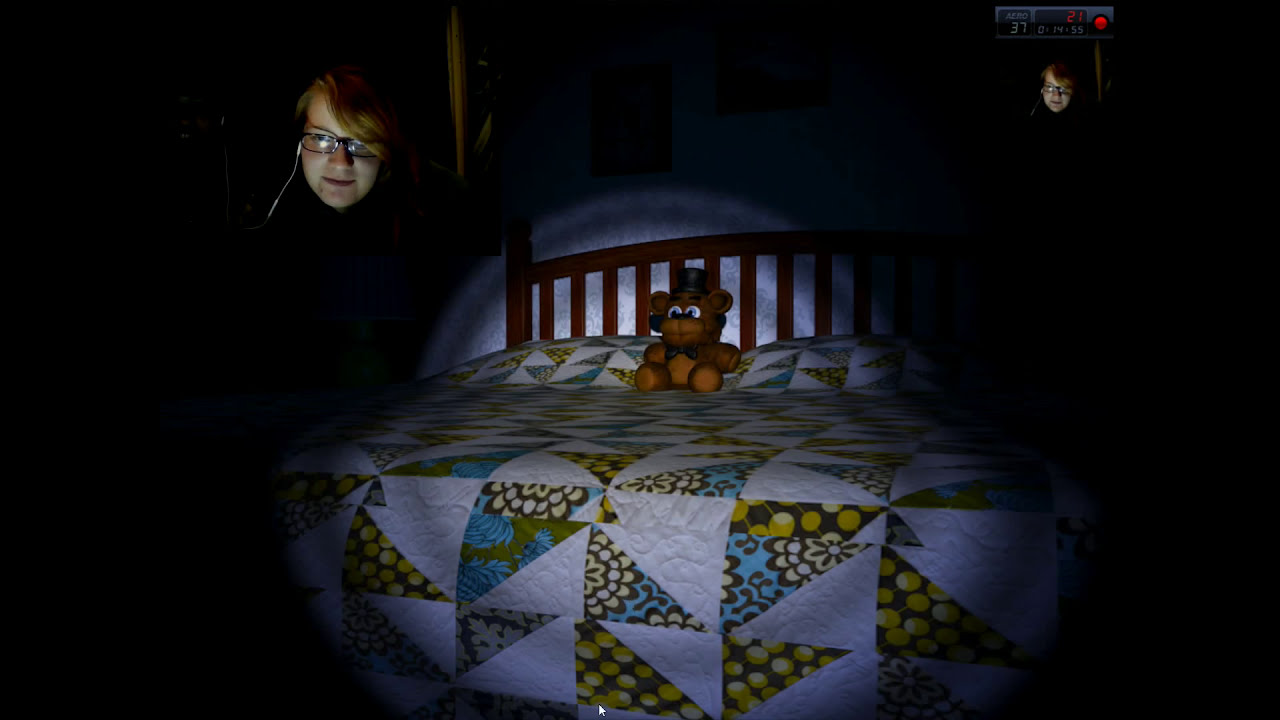The image is a dark, atmospheric screenshot from a video game stream, depicting a dimly lit bedroom with an eerie focus on a bed. The bed, centrally placed, features a geometric patterned blanket of squares divided into triangles, with some white squares adorned with green, yellow, and blue flowers. Positioned prominently on the bed, near the pillows, is a teddy bear with large white eyes staring directly forward, illuminated by a flashlight. The wooden headboard behind the bear has an arched top and vertical columns.

In the top left corner of the screen, there's a smaller overlay image of a young man wearing glasses with yellow lenses, slightly reminiscent of a video game streamer. Remarkably, a similar but smaller headshot of the same individual appears in the upper right corner. The left side of the image is dark, creating a stark contrast with the illuminated bed. The overall scene, bathed in darkness punctuated by the stark flashlight beam, suggests a spooky or horror game setting, highlighted by the eerie presence of the teddy bear and the subdued, haunting ambiance of the room.